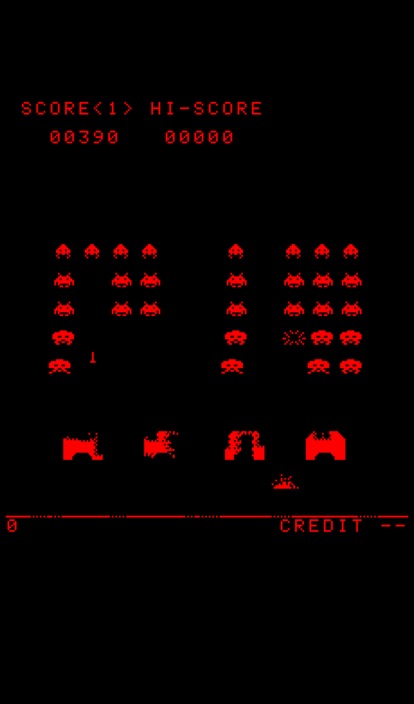The image is a vertically oriented rectangular screenshot from the classic video game, Space Invaders. The entire background is black, with all other elements in a striking red color. At the very top of the image, the text reads "SCORE < > HIGH-SCORE", with the score showing "00390" and the high score showing "00000". 

Beneath the score, there are eight columns of iconic alien invaders, neatly lined up, ready to descend. Four shield structures, resembling bunkers or hangars, are positioned below the columns of aliens. These shields serve as protection for the player's ship, which is located at the bottom of the screen.

Additional details include a horizontal red line below the shields, with the number "0" (possibly indicating the player's remaining lives) displayed to the left of the line. At the very bottom right of the image, the word "CREDIT" is clearly visible.